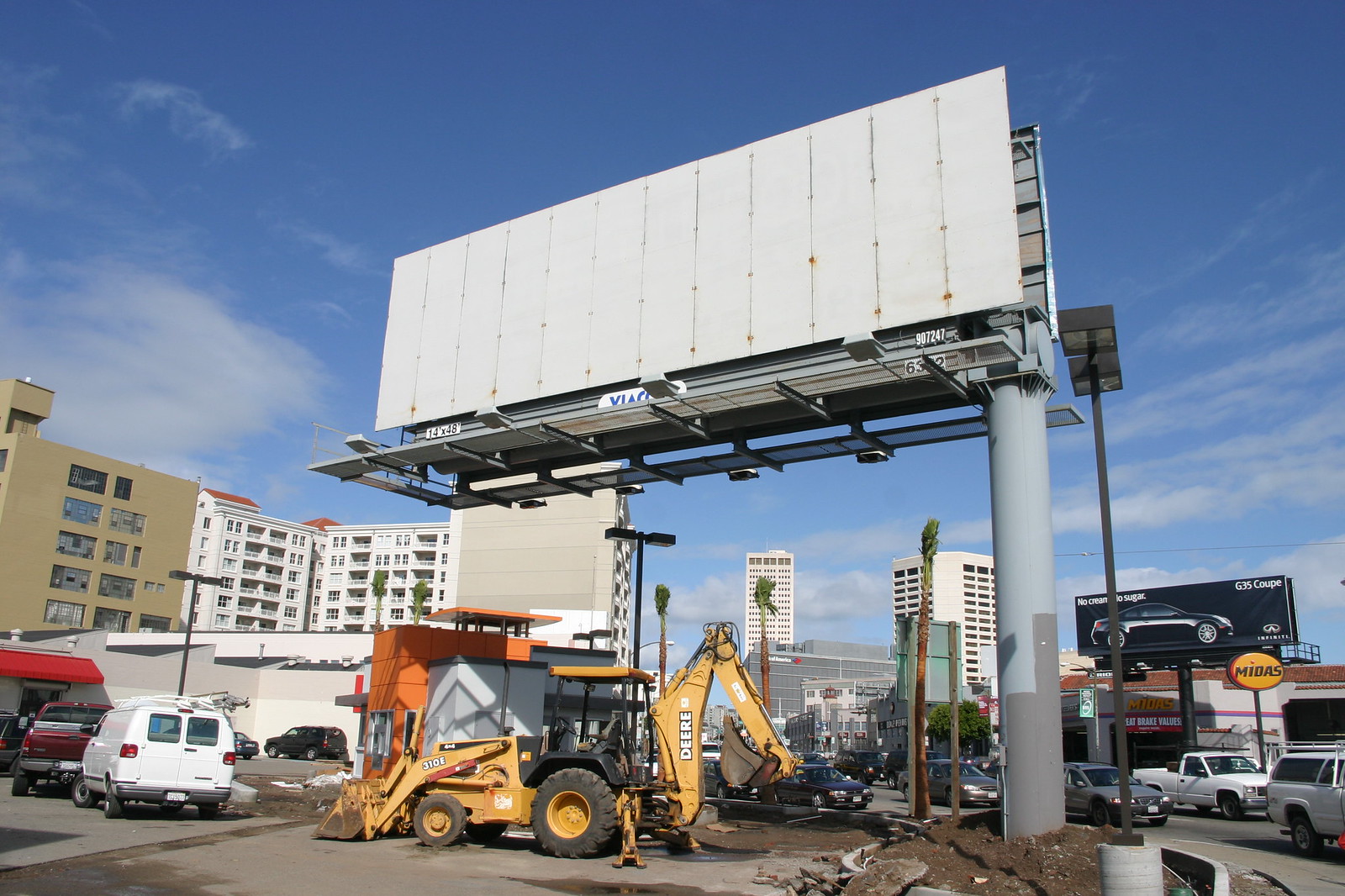The image portrays a bustling construction site bathed in daylight under clear, blue skies accented by dispersed, white clouds. On the left side of the frame, two tall buildings dominate the scene: one is white with numerous patios and a red roof, while the other is beige. Below, several vehicles are parked, including a red pickup truck, a white minivan with a silver ladder on its roof, and a red SUV. Prominent in the foreground, a John Deere excavator is actively digging into the black soil, creating a mound of disturbed earth. Overhead, an empty, slightly rusted billboard frame, with white panels and brown spots, stands as a silent witness to the ongoing construction activities.